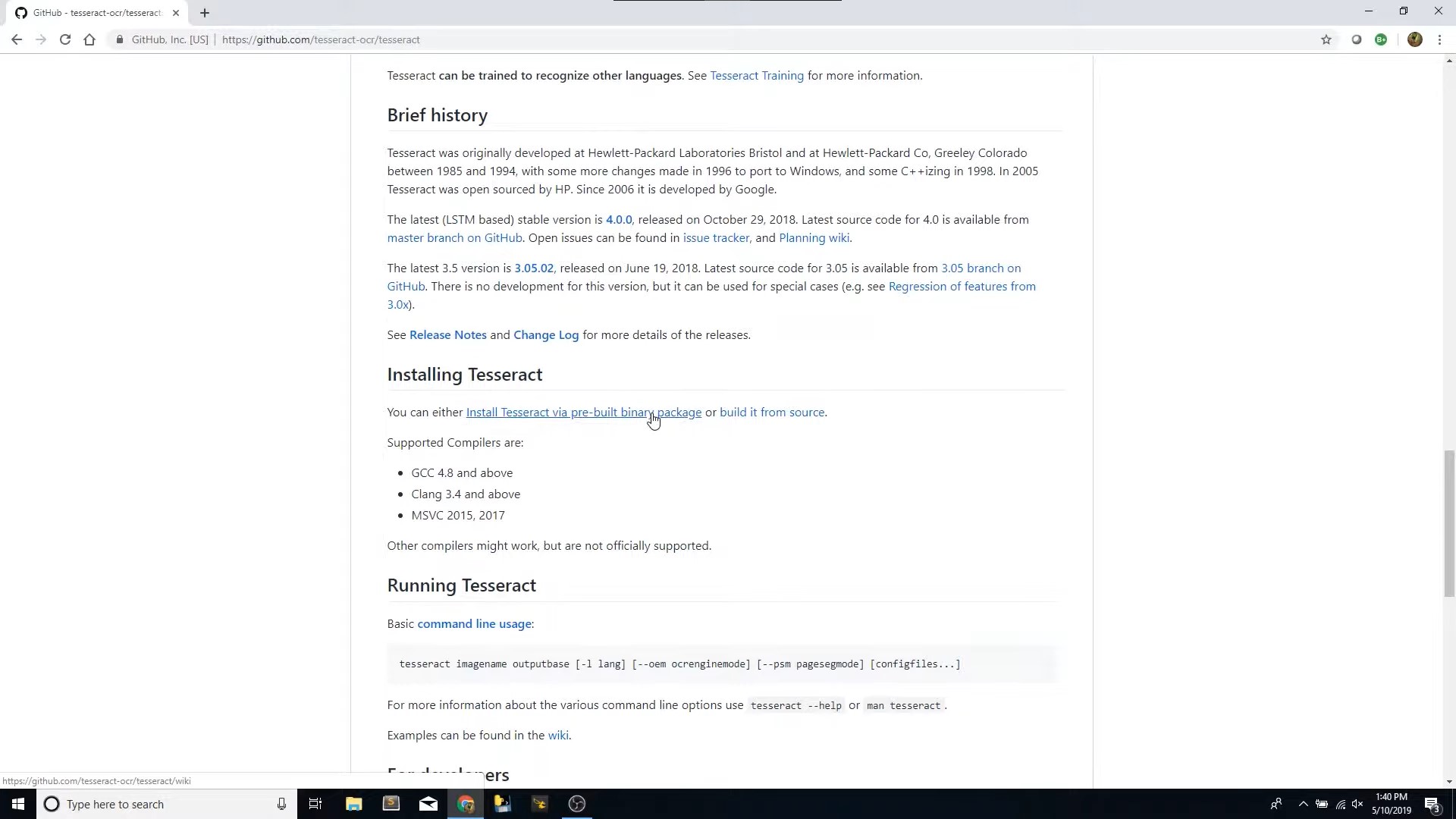The image contains a web page from GitHub. At the very top, there is a white tab with a black circular background on the left side, inside of which is the outline of a white cat. Next to the black circle, in black text, it reads "GitHub." Following that, there is a dashed sequence: "T-E-S-S-E-R-A-C-T dash O-C-R slash T-E-S-S-E-R-A-C-T," though the rest of the sequence is cut off. Beside it is a gray 'X' and a black plus sign, with the rest of the top section being gray.

Directly beneath this is a navigation bar containing several arrow icons (for back, forward, and refresh), a home symbol, and a gray oval with the text "GitHub, Inc." Inside brackets, there is "U-S-S-S-H-T-T-P-S" followed by "https://github.com/T-E-S-S-E-R-A-C-T dash O-C-R slash T-E-S-S-E-R-A-C-T."

The main content section begins with black text stating, "Tesseract can be trained to recognize other languages. See Tesseract for more information," where "Tesseract" is highlighted in blue. A section titled "Brief History" follows, detailing that Tesseract was originally developed at Hewlett Packard Laboratories in Bristol and Hewlett Packard Co in Greenland, Colorado, from 1985 to 1994. Additional changes were made in 1996 to port it to Windows, with some C++ modifications in 1998. 

The document further outlines that in 2005, Tesseract was open-sourced by HP, and since 2006, it has been developed by Google. The latest Long Short-Term Memory (LSTM)-based stable version, "4.0.0," released on October 28, 2018, is highlighted in blue. Source code for version 4.0 is available on the master branch on GitHub. The final section indicates that open issues can be tracked through the "issue tracker" and "planner wiki," both of which are hyperlinked in blue.